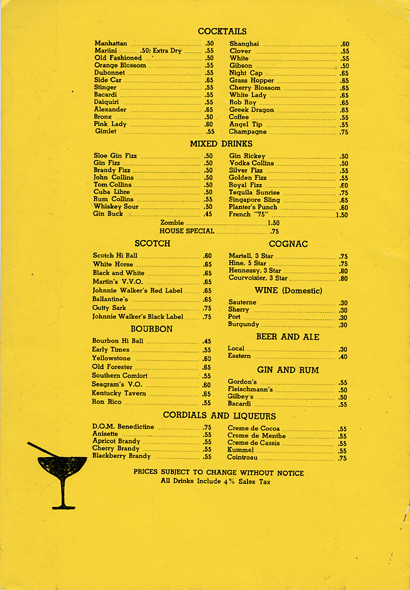The image features a detailed menu for a bar, elegantly printed with black lettering on a mustard-yellow rectangular paper. At the bottom left corner of the menu, a black martini glass with a little black stirrer sticking out to the side adds a touch of sophistication. The menu is organized into distinct sections, starting with "Cocktails," which lists a substantial variety of 26 different cocktails, although the specific names are not visible. Following that, there is a section for "Mixed Drinks," offering between 18 to 20 different options. The menu also boasts a diverse selection of spirits including 8 types of scotch, 4 types of cognac, 4 types of domestic wine, 8 types of bourbon, 2 types of barren ale, and 4 types each of gin and rum. Additionally, there are 10 types of cordials and liqueurs available. Notably, the prices on the menu are subject to change without notice, and all drink prices include a 4% sales tax. The layout is clean and straightforward, with no other wording or imagery present on the page aside from the martini glass graphic.